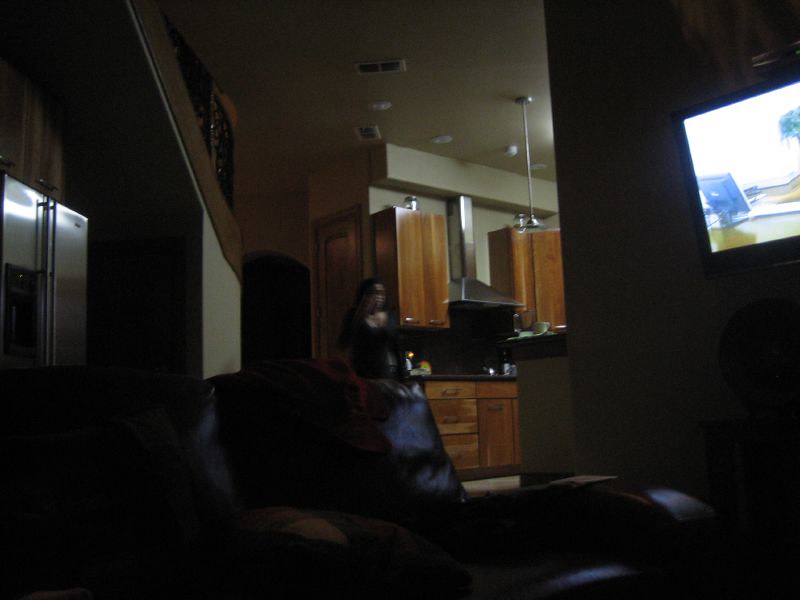The photograph captures the interior of a house from the perspective of a darkened living room, looking into a brightly lit, modern kitchen. The living room and kitchen are connected by an open floor plan with no doors separating the two areas. A black leather armchair is positioned at the bottom center of the image, slightly leaning back towards the left. The focal point in the living room is a television in the upper right corner, displaying what appears to be an outdoor scene. In the kitchen, a large silver double-sided American-style refrigerator stands prominently on the left. The kitchen features brown cabinetry, shiny silver light fixtures, and an overhead stainless steel hood above the stove. The beige ceiling has recessed lighting that illuminates the space. Centrally, a woman with long brown hair, wearing a scoop neck top, is captured walking towards the kitchen, creating a sense of motion in the otherwise still composition.